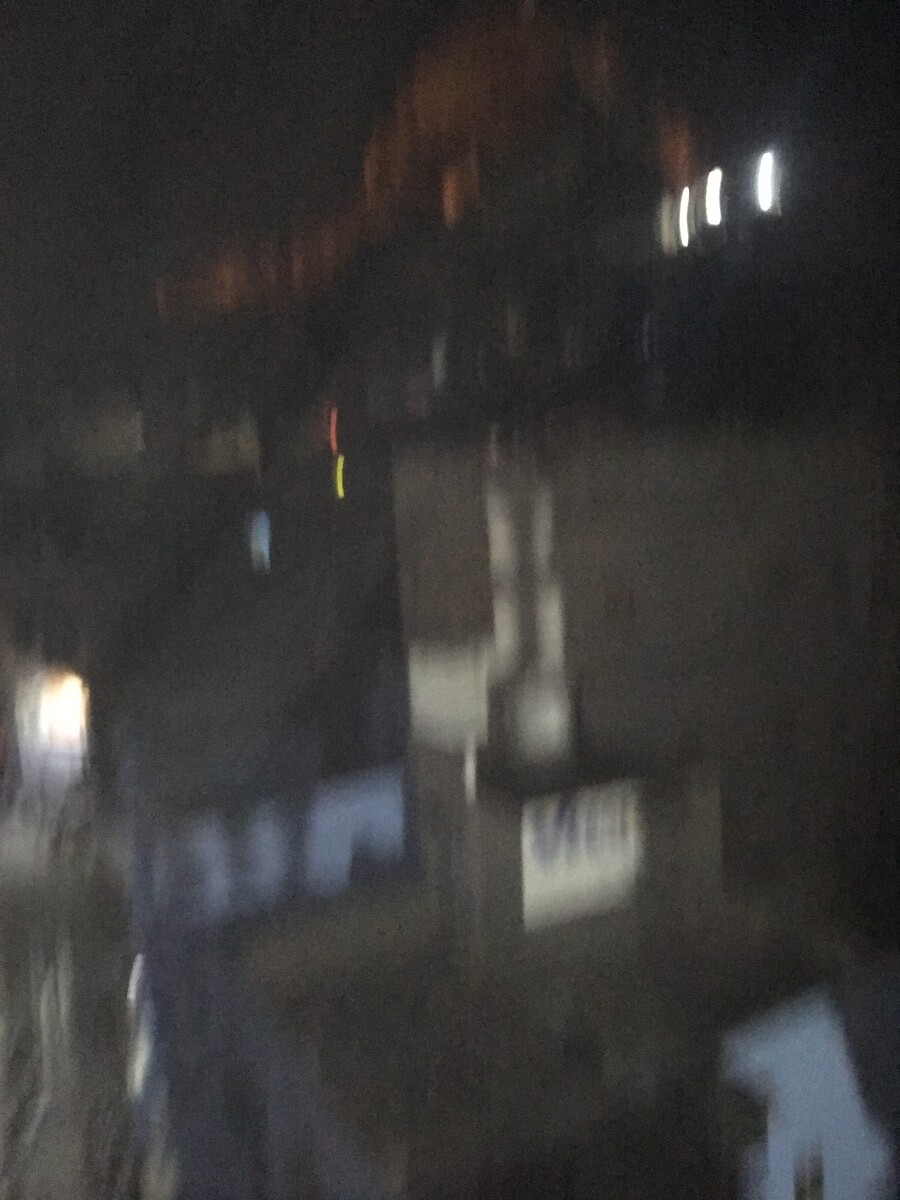This image appears to have been taken at night and is extremely blurry, making it difficult to discern precise details. It seems to capture a scene of an urban area, potentially an Italian town on a hillside, as viewed from above. Dominating the image is a large concrete building with multiple levels and numerous windows, possibly a motel or hospital. A white sign with blue letters, potentially reading "MGI," is visible on this building. The surroundings include scattered lights from various sources, including windows and street lamps, which illuminate parts of the scene. In the lower right, there appears to be a smaller white house with a black roof. Overall, the combination of night-time darkness and the blurry quality gives the impression of a hasty, possibly inebriated snapshot.